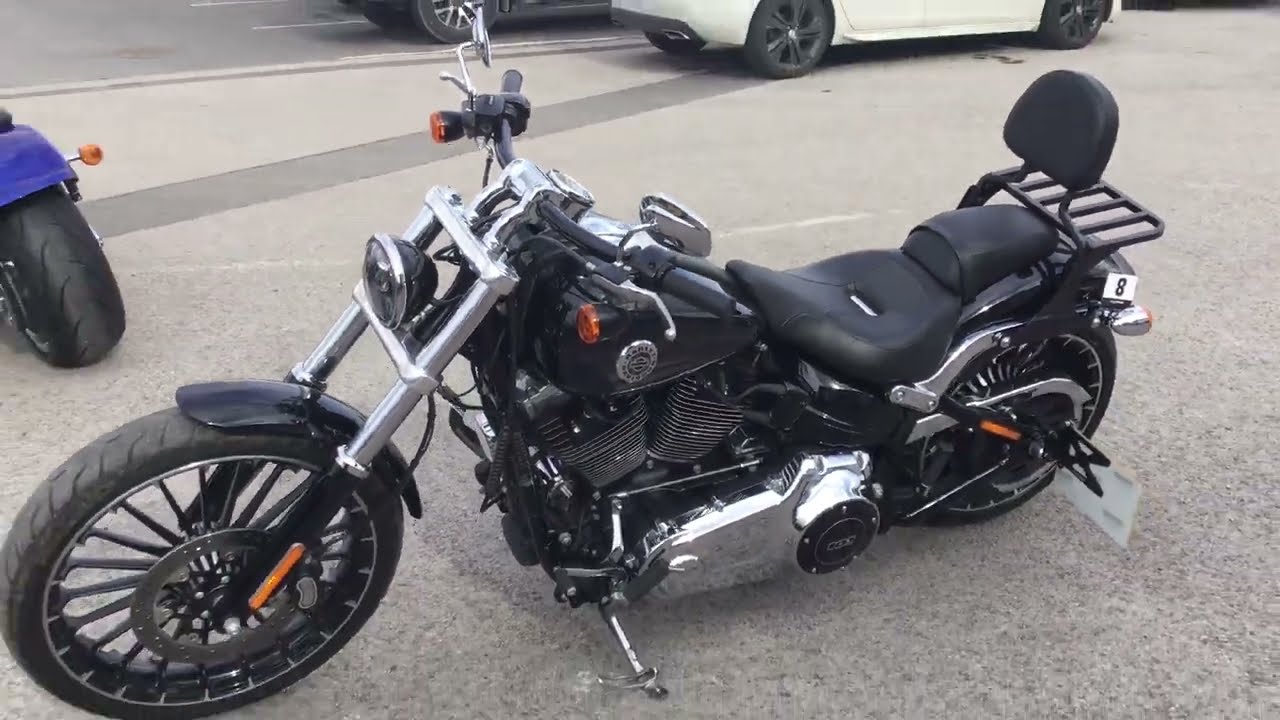The photo captures a sleek, black motorcycle parked on a street during the daytime. The bike features a shiny silver or stainless steel frame, with black components including the gas tank, fenders, seats, handlebars, and tires. The crankcase and some front parts of the motorcycle are also silver, adding to its polished appearance. The kickstand is deployed, indicating that the motorcycle is stationary and unoccupied. Prominently displayed on the rear of the motorcycle is a small, white card with the black number 8.

In the left-hand side of the image, a portion of another motorcycle with a distinctive blue fender can be seen. Additionally, a white car and parts of other vehicles are visible behind the black motorcycle, suggesting the bikes are parked by the roadside. The photo is high-quality and taken in bright, clear natural light, emphasizing the motorcycle's well-maintained and polished condition.